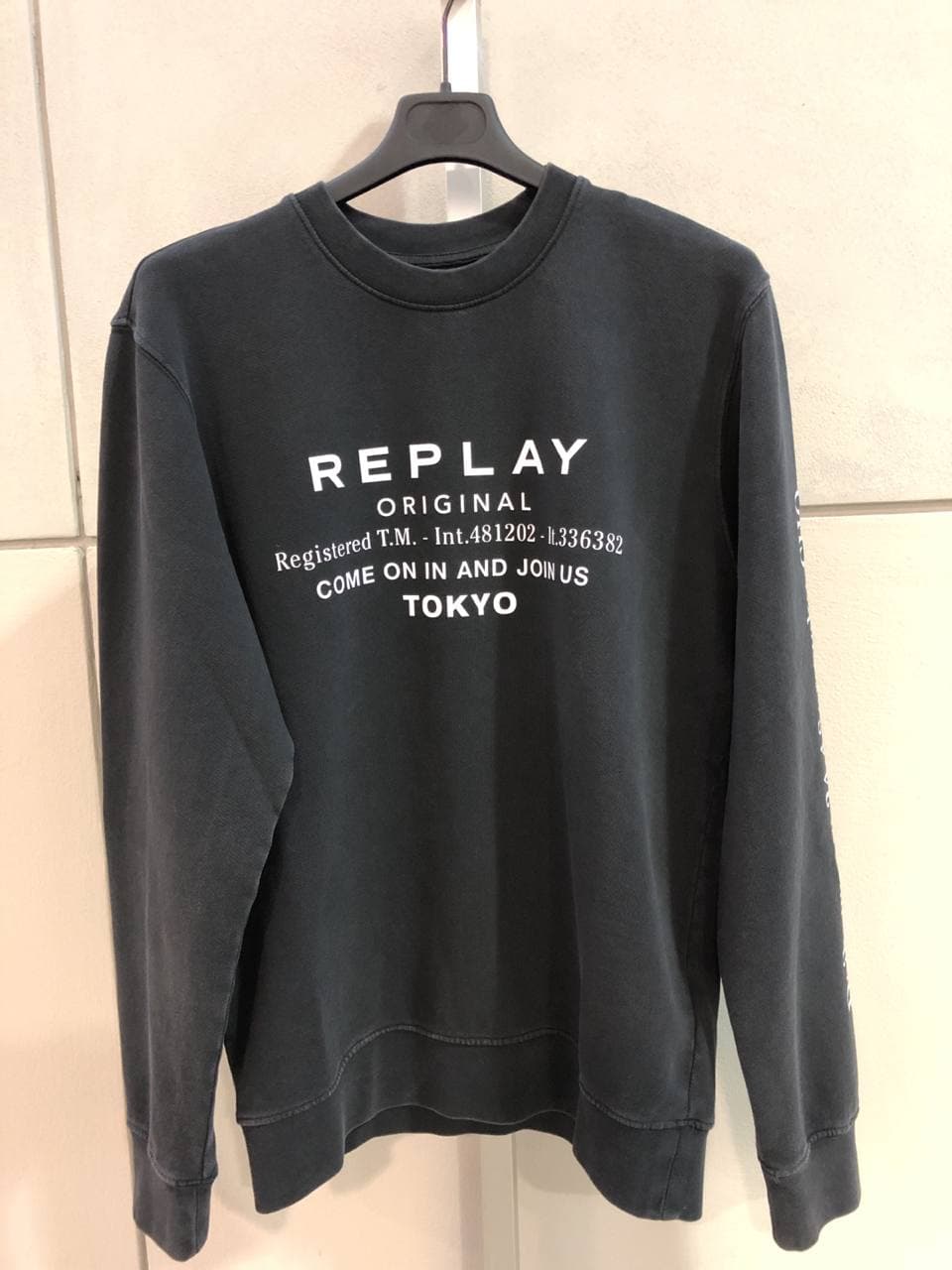This photograph prominently features a black, long-sleeve crew neck sweatshirt hanging on a black plastic hanger with a metal hook, centered against a wall composed of large light pink tiles with gray grouting. The sweatshirt, loose and with its sleeves hanging straight down, displays prominent white text on the chest. The largest text reads "REPLAY ORIGINAL" in a sans-serif font. Below this, in smaller serif font, is "REGISTERED TM INT 481202 LT 336382," followed by "COME ON IN AND JOIN US" in sans-serif, and finally "TOKYO" in bold sans-serif font at the bottom. The sweatshirt also has ribbing along the cuffs of the wrists and the hem at the bottom, adding to its detailed appearance. The setting suggests a minimalistic backdrop, potentially indicative of a clothing store or a styled home interior.